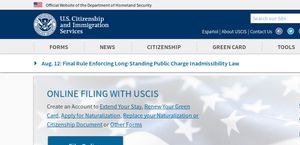This image features a webpage for the U.S. Citizenship and Immigration Services (USCIS). Dominating the top left corner of the page is an indistinguishable logo, followed by a prominently placed search box on the right. Directly beneath the logo and search box is a navigation menu with three tabs, including "Contact Us," and social media icons for sharing and following on Facebook and Twitter. Further below, an additional set of tabs is visible, categorized as "Forms," "News," "Citizenship," "Green Card," and "Tools."

The main body of the webpage displays a faint backdrop of the American flag. Superimposed over the flag is text promoting online filing through USCIS, accompanied by several hyperlinks. These links appear to read "Extend Your Stay," "Review Your Green Card Application," "Naturalization," and possibly references to citizenship documents or other forms. The comprehensive layout effectively guides users through the varied resources and services offered by USCIS.